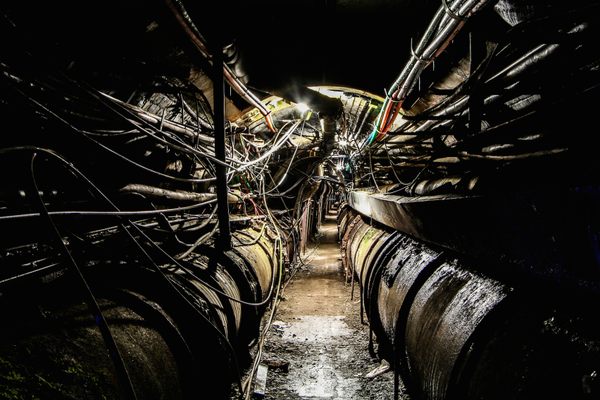The image depicts the dark, confined interior of what appears to be an industrial facility or possibly an underground tunnel. The setting is ominous, with a narrow hallway featuring a rounded ceiling, allowing moisture to seep through, creating glossy patches on the floor where water has pooled into mud. The walls on both sides are lined with large cylindrical drum tubes and an intricate network of pipes. Miles of tangled cables, in varying colors such as white, black, and orange, as well as numerous hoses, either trailing or patched together, drape haphazardly across the scene. This network of cables and hoses stretches far into the distance, contributing to the chaotic and foreboding atmosphere. The setting's dim lighting, punctuated by a few scattered light bulbs, further enhances the eerie, almost dystopian vibe, reminiscent of the interior of a monstrous machine or the organs and vessels of a demonic creature.